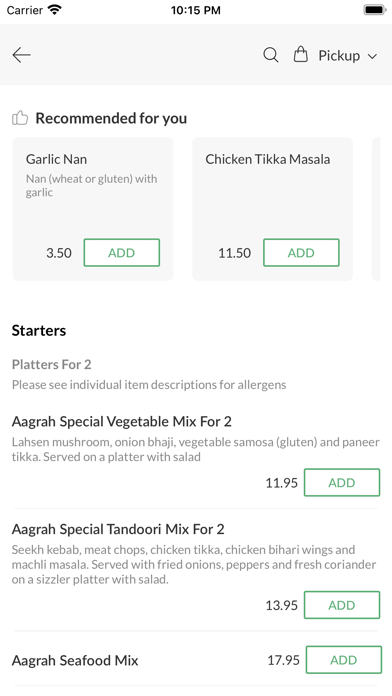**Screenshot of Mobile Phone Application**

The screenshot displays a mobile phone application interface. At the very top, there is a white header containing various black icons. Directly below, a light gray header is visible. The far left of this header features a dark gray left-pointing arrow. Progressing to the right, the icons include a dark gray magnifying glass, a dark gray shopping bag, dark gray text stating "Pickup," and a dark gray downward-pointing arrow.

Beneath this, in the top left corner, a light gray thumbs-up icon is present. Adjacent to this icon, bold black text reads "Recommended for you." Below this recommendation section, there are two light gray rectangular panes with rounded corners, each displaying detailed information.

The first pane lists the item "Garlic Naan" in bold dark gray text at the top left. Below this, in smaller light gray text, "Naan (wheat or gluten)" is written, followed by "with garlic." Centered beneath this description, the price "$3.50" is written in black text. To the right of the price, there is a white rectangle with a green outline, containing green all-caps text that reads "ADD."

The second pane follows a similar layout, with "Chicken Tikka Masala" in bold dark gray text at the top left. The price "$11.50" is centered beneath the description, and to the right, another white rectangle with a green outline contains the green all-caps text "ADD."

Further down, after a small area of negative space, the top left corner displays bold black text that reads "Starters." Below this headline, medium gray text states "Platters for two." Further down, smaller light gray text advises, "Please see individual item descriptions for allergens."

Below this advisory, black text introduces the item "Agra Special Vegetable Mix for Two." The description includes light gray text listing "Lasan Mushroom, Onion Bhaji, Vegetable Samosa (gluten), and Paneer Tikka served on a platter with salad."